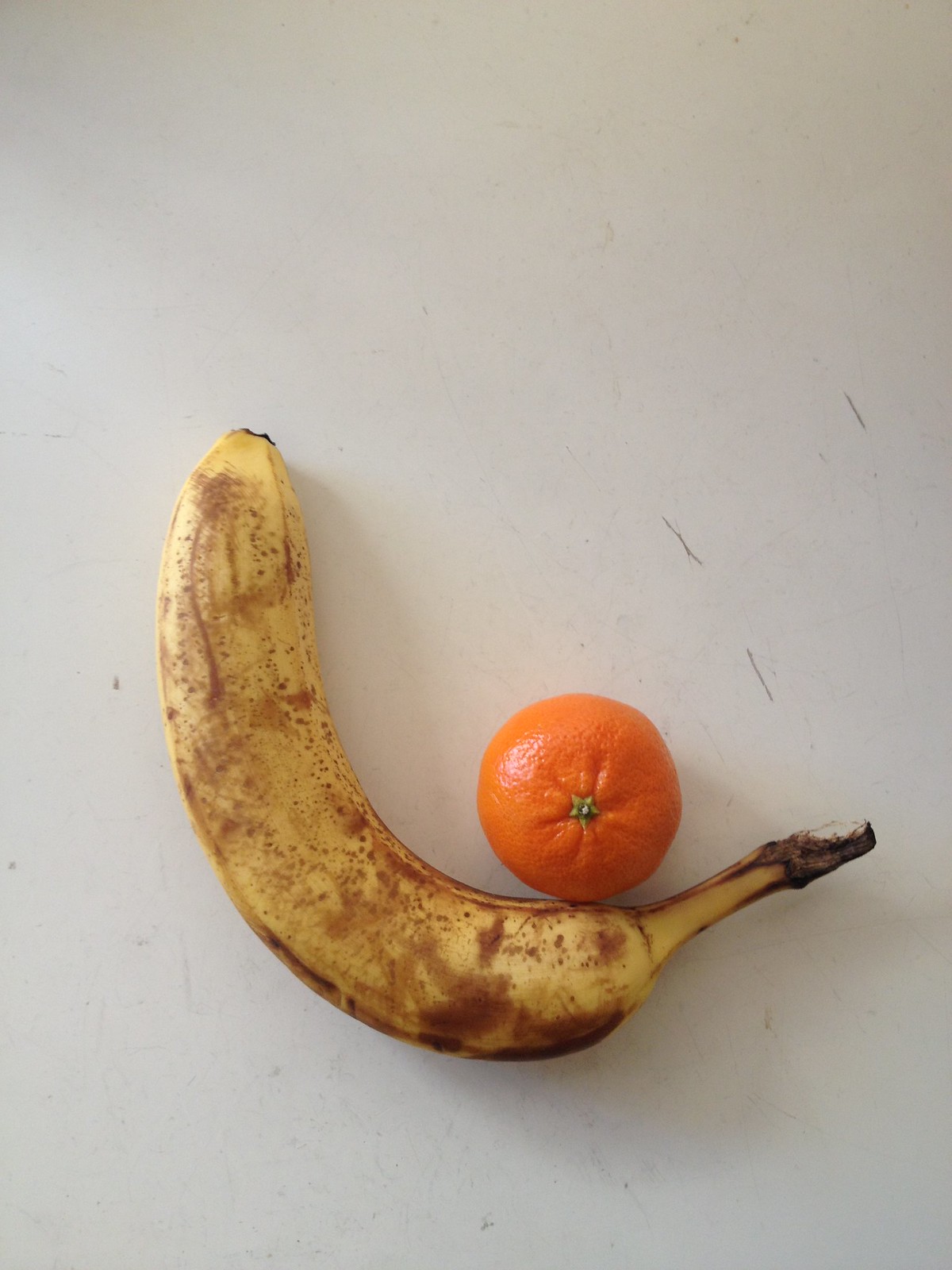The photograph features a rectangular composition where the width is twice the height. Set on a flat, white-painted surface marred with scratch marks and cuts revealing the light brown to gray wood underneath, the image captures a single banana and an orange. The banana, displaying signs of aging with brown spots along its yellow skin, has a blackened stem and a darkened patch at the bottom end. It is positioned with its curved side facing downwards, pointing towards the bottom left corner, while its stem reaches towards the center right. Next to the banana's stem sits the vividly orange-colored fruit. The orange's upper left side is slightly reflective, indicating a light source, and it features a green, five-pointed star-shaped stem at its center.